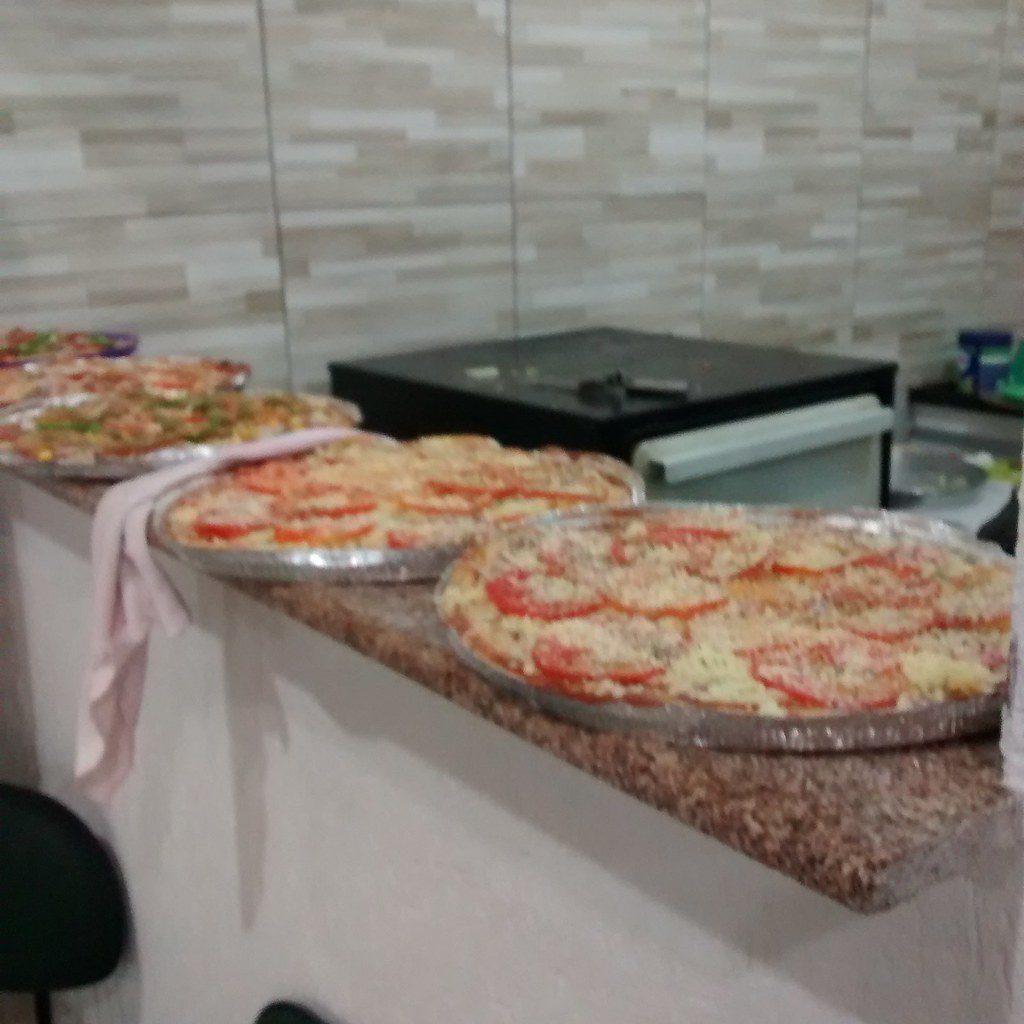In this color photograph, a well-lit kitchen scene showcases a high bar-level granite countertop featuring four round, uncooked pizzas resting in aluminum trays. The countertop, a rich brown with various lighter and darker brown flecks, holds the pizzas in a neat row extending from front to back. The first two pizzas prominently display shredded cheese and tomato slices, while the third pizza in the background appears to have additional green and black toppings. The fourth pizza is partially obscured and less distinguishable.

A pink rag is positioned behind the second pizza from the front, draping slightly over the side. To the right of the pizzas, a small black-and-gray portable oven sits against a white wall, its door slightly ajar. The kitchen walls behind the counter are adorned with evenly sized square tiles, each patterned with horizontal rectangular strokes in varying shades of gray and beige. Below the countertop, white cabinetry is visible, and a blue box rests atop another cabinet nearby. A bar stool or two are partially pushed under the counter, adding a casual element to the space. The entire scene is bathed in a natural, warm light, emphasizing the textures and colors throughout the kitchen.